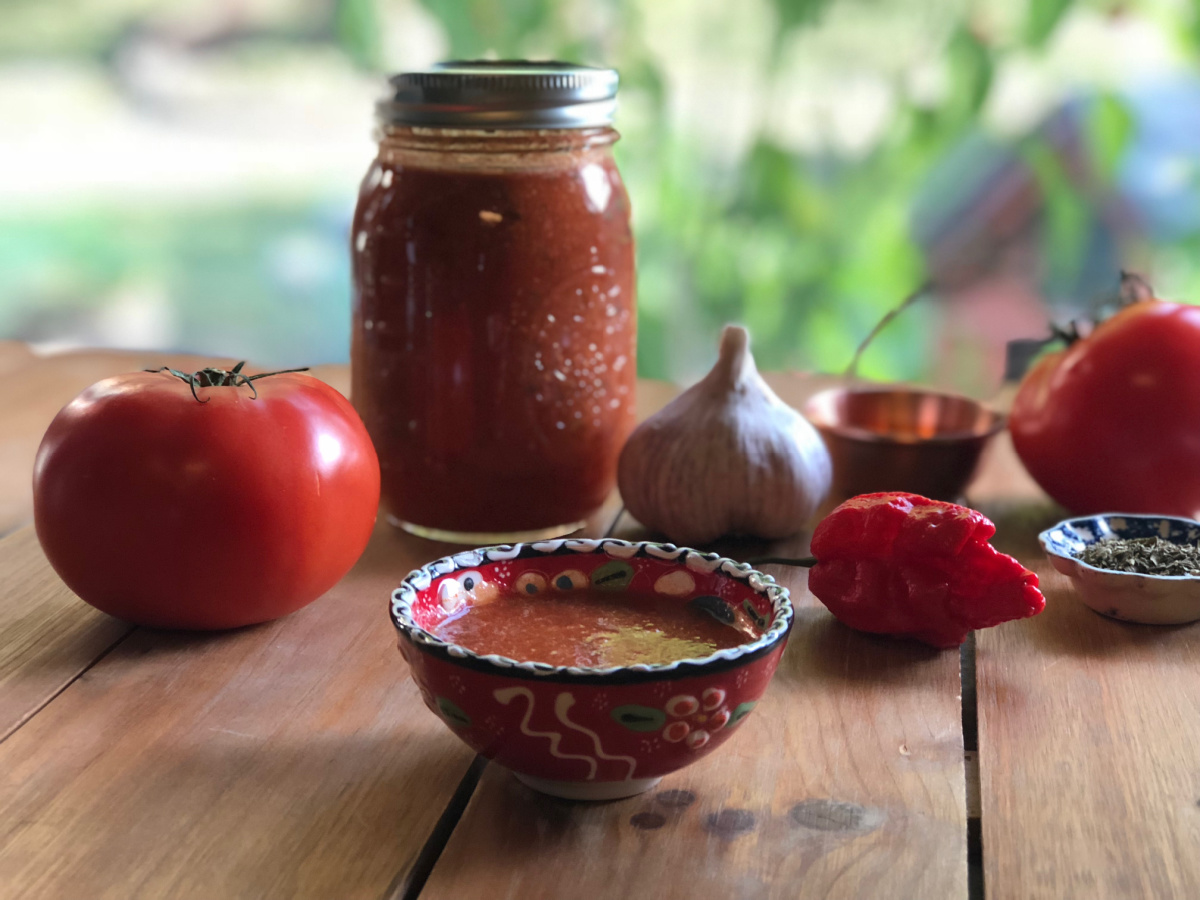This image captures an idyllic outdoor scene centered around a beautifully decorated, clay bowl of vibrant salsa. The bowl, a striking red adorned with intricate designs of berries, leaves, and white squiggly lines, features a black and white rim. It is prominently placed on a wooden picnic table with visible wooden slats, enhancing the rustic charm of the snapshot. To the left of the bowl lies a ripe tomato, while a fiery red chili pepper sits to the right. Behind the bowl, a whole bulb of garlic adds to the array of fresh ingredients, alongside a glass jar with a metal twist top, unmistakably filled with the same salsa as in the bowl. To the further right, a smaller bowl filled with black seeds complements the composition. The background is softly blurred, hinting at flourishing plants and a railing, affirming that the photo was taken in an outdoor setting, focusing on fresh, garden-to-table simplicity.